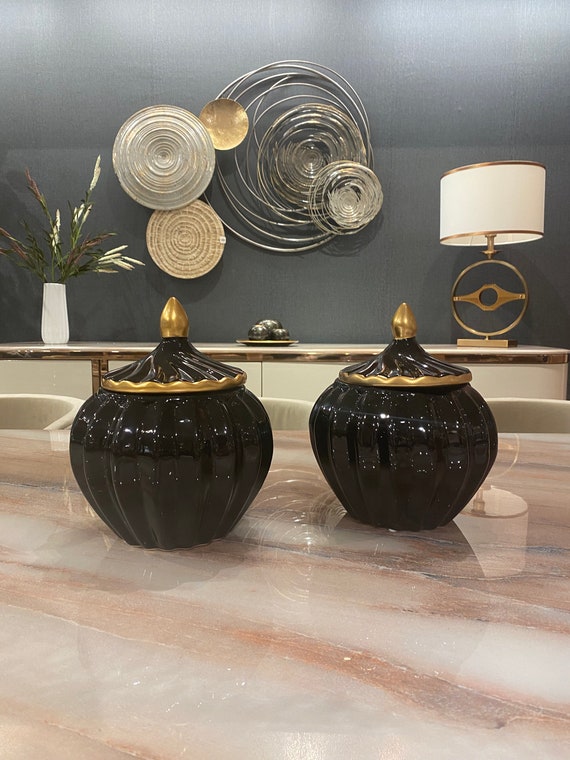The photograph showcases two black jars with a glossy finish, resembling pumpkins due to their grooved design, situated prominently on a white marble tabletop streaked with light orange. Each jar possesses a gold-rimmed lid with a dome-shaped gold handle. The tabletop, which exudes luxury with its pristine and shiny surface, sits in front of modern chairs pushed against it. In the background, a beautifully designed decor scene includes a lamp with a white lampshade and a gold body, a white vase containing dried flowers, and a small plate holding three black decorative balls. The backdrop features a sophisticated wall painted in gray and adorned with interwoven circular metal designs in silver and light gold, reinforcing the image's upscale and artistic ambiance.